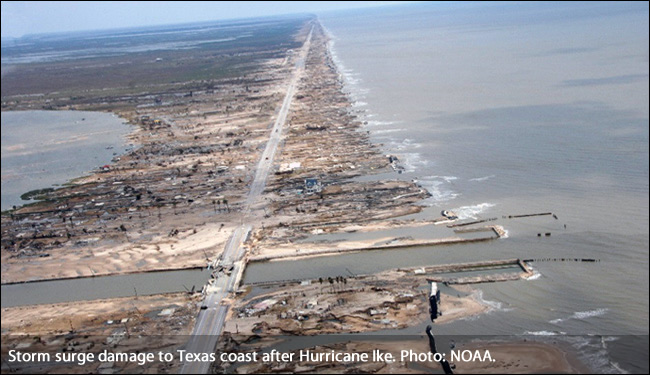This aerial photograph depicts the extensive storm surge damage to the Texas coast after Hurricane Ike, as captured by NOAA. The scene reveals a coastal landscape ravaged by the hurricane, with a muddy, disheveled beach area flanked by water on both the left and right. A long, damaged road runs through the center, partially washed out and covered in debris, with stranded vehicles visible on its surface. The land appears largely barren in parts, while patches of dark brown and light brown sand intermittently show through the scattered debris and shallow water. In the upper left, the sky or a blue-toned section of the image can be seen. The caption at the bottom left of the image reads: "Storm surge damage to Texas coast after Hurricane Ike. Photo: NOAA."